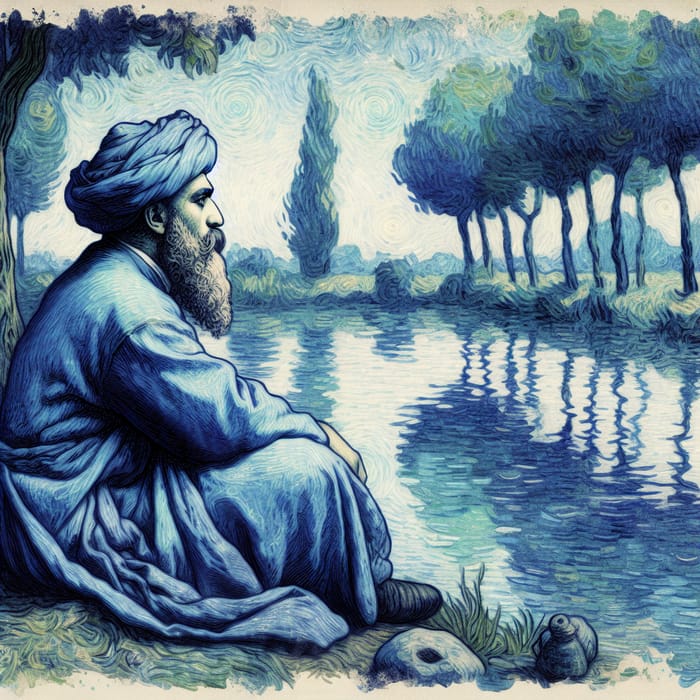This painting, evocative of Vincent van Gogh's distinctive style, vividly portrays a contemplative Middle Eastern man seated by a pond. Dominating the left side of the canvas, the man's dignified presence is accentuated by his flowing blue robe and a matching curled-up scarf or Magi hat. His long beard, streaked with shades of white and dark gray, alongside his black shoes, enhances the air of mysticism surrounding him. He gazes thoughtfully to the right, seemingly lost in contemplation. By his side, a sturdy rock and a vessel, likely for holding drinks, add further layers of narrative to the scene.

The background bursts with dynamic, swirling brushstrokes characteristic of Van Gogh, with the upward spiraling trees and a sky rendered in starry-night blues and whites. The entire composition weaves together hues of blue, green, and gray, creating a harmonious yet vibrant palette. The trees’ reflections dance in the river’s surface, mimicking the same swirling patterns seen throughout the piece. Further in the distance, a hint of rolling hills can be discerned, adding depth and context to this serene moment captured in paint.